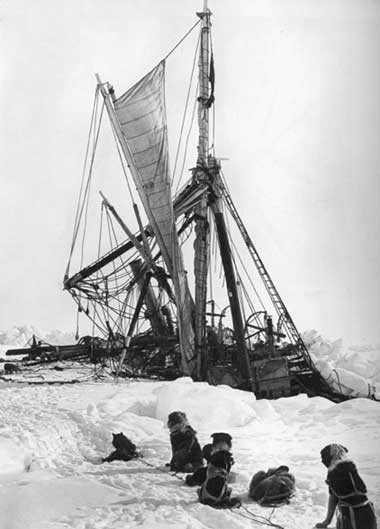The black and white photograph captures a snowy, desolate landscape featuring a group of sled dogs and a partially sunken ship. Several dogs, adorned with harnesses, are positioned in the snow; one in the bottom right corner sits upright, showcasing a white neck and a harness that wraps around its chest. Another dog lies flat on the ground while the rest either sit or lie down in various positions, with one having noticeable black and gray patches. The dogs appear to be connected by harnesses and ropes, indicative of a sled team.

In the center of the image, a ship is prominently visible, buried up to its deck in snow and ice, suggesting it's immobilized. The ship’s masts are collapsed and poles jut out in various directions, supported by a network of wires. A partially unfurled sail and scattered rigging add to the ship’s forlorn appearance. The background is a featureless expanse of solid white sky, emphasizing the isolation and harsh conditions likely faced during a polar expedition. The ground appears disturbed, with steps and tracks suggesting movement around the area. In addition to the dogs, a packet or bundle lies on the snow, contributing to the sense of an abandoned or ongoing expedition.